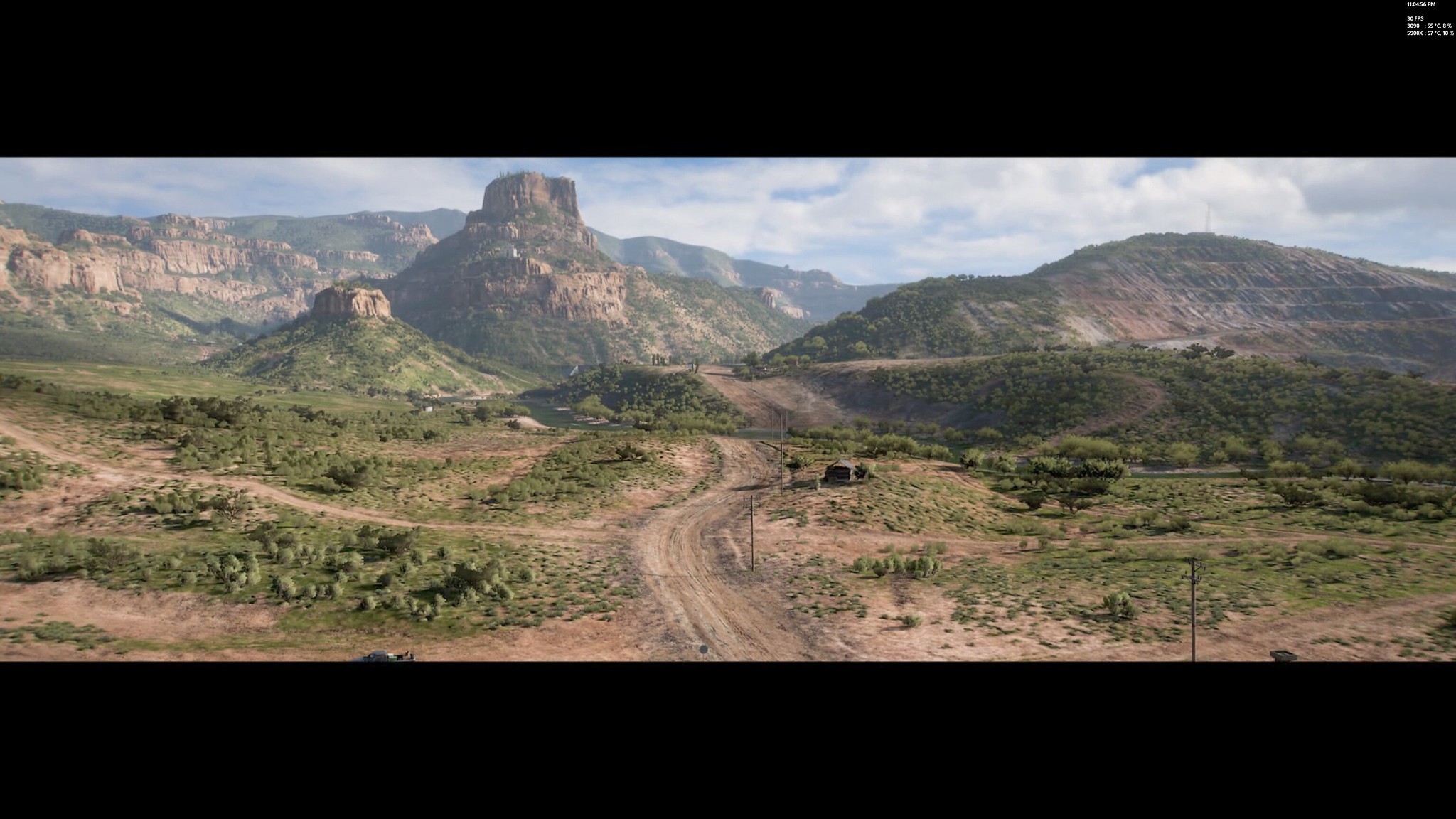A computer-generated image, likely from a video game, features a panoramic scene framed with black bands at the top and bottom. The sky is a serene light blue with scattered white clouds. In the background, distant mountains in shades of gray and tan provide a striking contrast. Closer to the center, more gray and tan mountains rise prominently. The image is dominated by a winding dirt road that begins in the forefront, meandering over a small hill and through the mountainous landscape. This main road splits into various paths—one diverging to the right and another to the left, with a couple more branching off in the forefront. While the dirt road boasts a realistic texture, some of the green bushes scattered along the scene appear noticeably artificial.